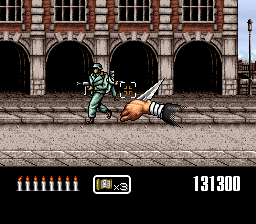This is a detailed screenshot from an old 1990s era video game, presenting classic retro pixel graphics. The scene appears to be a first-person perspective, with the player's hand gripping a large dagger prominently displayed. Opposing the player's hand is a green-uniformed soldier, complete with a military helmet and holding a gun. The background setting features an industrial or antiquated town atmosphere, potentially reminiscent of Germany, with prominent architectural elements like big black archways and red color accents.

About 80% of the screen is dedicated to the gameplay, depicting a concrete road flanked by paving slabs which suggest pavements, and a grand building in the distance. The bottom quarter of the screen is a black background menu displaying critical game stats: 

- On the left side, there are 8 bullet indicators, resembling small white candles or shotgun shells.
- The middle section shows a white flag icon with a "x3," likely indicating three lives remaining.
- On the right side, the player's score is prominently displayed as 131,300.

Additionally, hovering over the gameplay area, there's an icon representing a hand holding a dagger, possibly serving as the game’s cursor or a targeting indicator. Overall, this screenshot provides a rich, nostalgic snapshot of an intense action sequence from a classic platform fighting game with a possible military or combat theme.